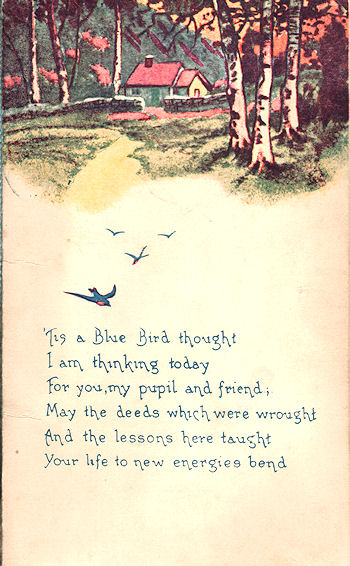The image depicts an artistic greeting card set on pinkish paper. At the top, a detailed drawing showcases a picturesque scene featuring a house with a red roof and green door, surrounded by various natural elements. In the background, a range of mountains stretches out under a pink sky, while trees adorned with pink and white blossoms add to the whimsical landscape. A concrete foundation encircles the house, which is further enclosed by a barricade. In front of the house, hedges with an opening are visible, and in the foreground, trails wind through patches of grass.

The card is further embellished with four birds soaring above, three small ones at the forefront, and one larger bird slightly to the left. Below this serene illustration, a poem is elegantly printed in blue ink: 

"'Tis a blue bird thought I am thinking today for you, my pupil and friend, may the deeds which were wrought and the lessons here taught your life to new energies bend."

The bottom of the card retains its simple pink hue, providing a subtle contrast to the detailed imagery and meaningful text above.